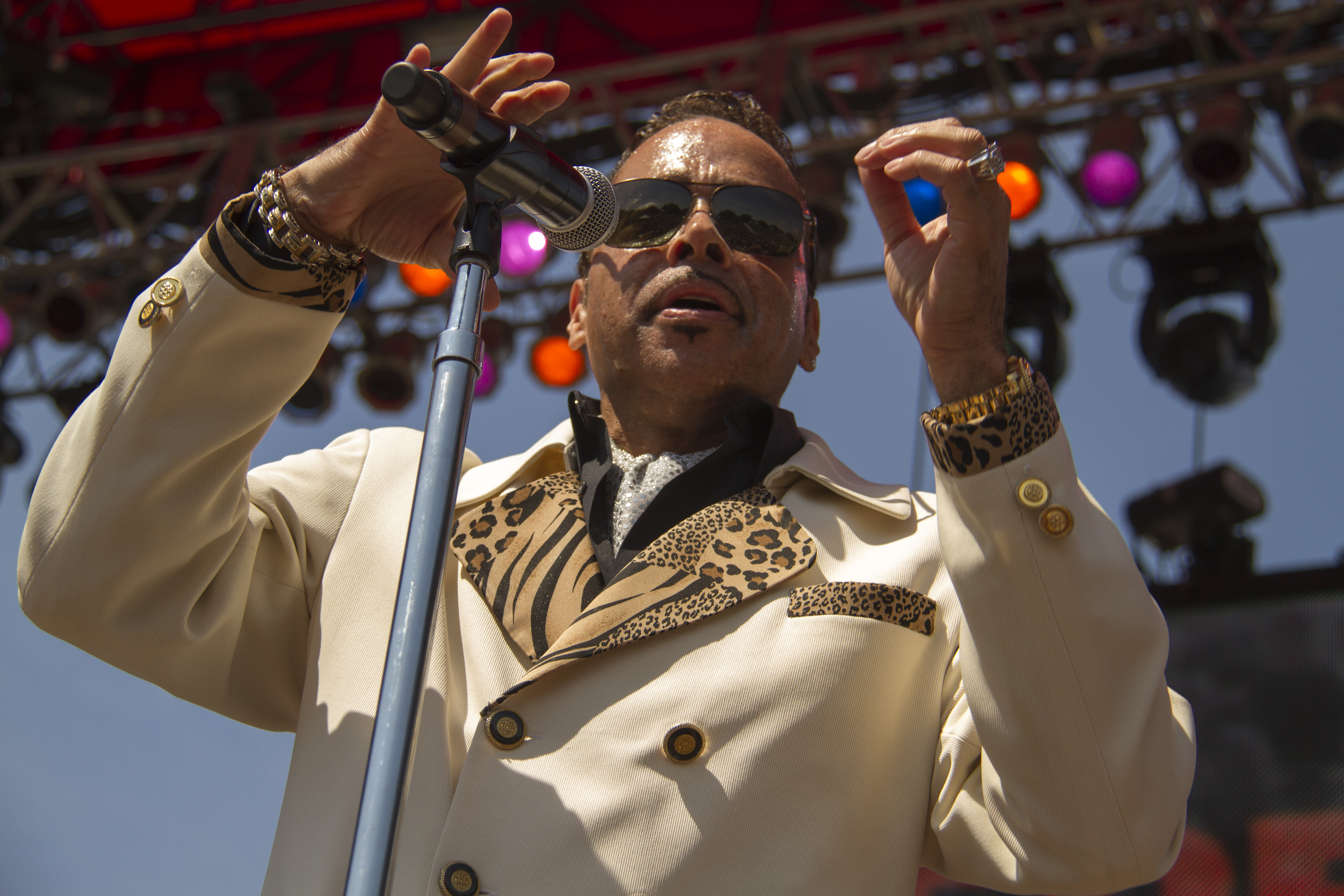The image captures Morris Day standing confidently on a stage, viewed from a lower angle that emphasizes his commanding presence. He is in front of a black microphone mounted on a long, silver stand. Morris is dressed in a striking light yellowish-beige suit adorned with distinctive cheetah print accents around the collar, pocket, and wrists. Underneath the suit, he sports a black dress shirt complemented by a white neckerchief, adding a touch of elegance. His look is further accentuated by an oversized pair of sunglasses, a pencil-style mustache, and a small soul patch. Both of his wrists are adorned with thick bracelets or watches, and a prominent ring sparkles on his left hand. His hands lightly rest over the microphone, suggesting a moment of pause or anticipation. In the background, myriad colored stage lights illuminate the scene, framing Morris against a backdrop of a blue sky, indicating an outdoor performance. The golden buttons on his suit and the silver sequined necktie add a final flourish to his dazzling stage ensemble.